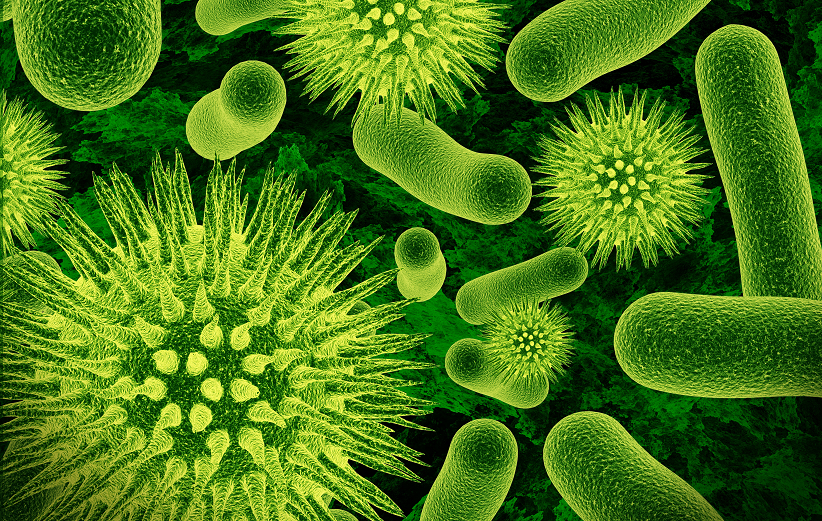The image features a striking, neon yellow-green color palette set against a stark black background, creating a vivid and eye-catching contrast. The composition appears to be a digital or AI-created artwork, reminiscent of microscopic views of bacteria or viruses. Prominent in the image are spiky, spherical forms that evoke the look of exaggerated germs or even COVID-19 particles, with textures that resemble spiky earrings one might find at trendy stores like Hot Topic or Claire's. Accompanying these are long, see-through, tubular shapes suggestive of amoebas or parasites, adding to the organic and somewhat unsettling feel. The image's various elements, from the spiky orbs to the liquid-like tubes, all appear wet and glossy, contributing to a sensory-rich visual experience. The backdrop includes subtle smudges, enhancing the organic, microscopic aesthetic. The shades of green range from a light, almost yellow hue to very dark green, almost merging with the black background, further heightening the dramatic impact of the artwork.